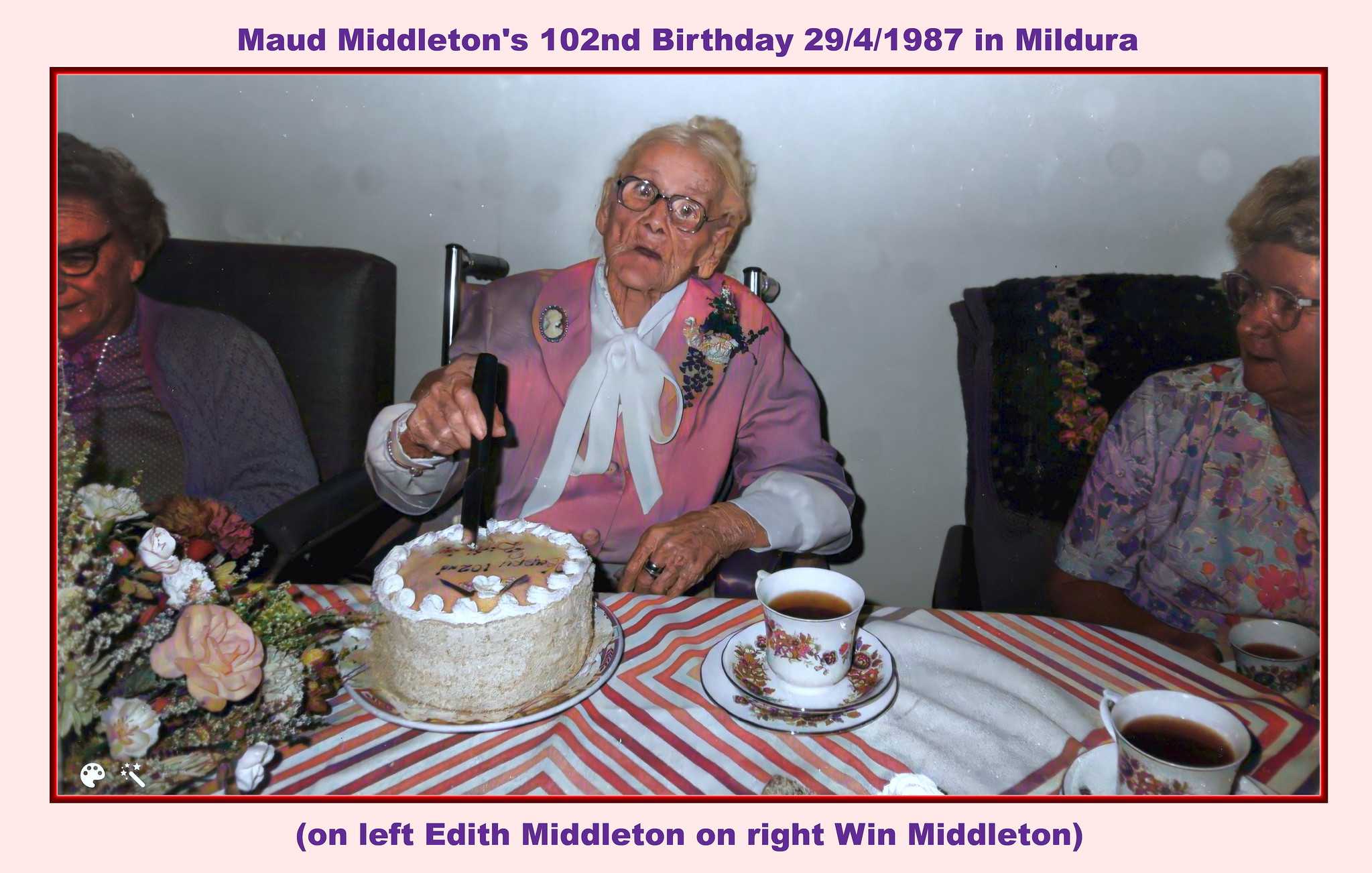This is a photograph capturing the 102nd birthday celebration of Maude Middleton, taken on April 29, 1987, in Mildura. The image features three elderly women, identified from left to right as Edith Middleton, Maude Middleton, and Wynne Middleton. 

Above the photograph, the text reads "Maude Middleton's 102nd birthday, 29-4-1987 in Mildura." Below the photo, the names are annotated with "on left, Edith Middleton," and "on right, Wynne Middleton."

Maude, positioned at the center, is the focal point and is seen cutting into a birthday cake with a knife held in her right hand. She has white hair and is wearing black glasses. Her attire includes a pink jacket over a white shirt, accented with a white ribbon at the neck, a brooch on her right lapel, and a corsage on her left lapel. A glass of tea rests on a saucer in front of her.

Edith Middleton, seated on the left, is dressed in a gray sweater over a gray shirt, accessorized with a strand of pearls. Wynne Middleton, on the right, is depicted sitting in a gray chair with an afghan draped over the back. She wears a floral short-sleeve shirt and also has a cup of tea in front of her. Both Edith and Wynne are wearing glasses and appear to be looking towards the cake that Maude is cutting. This intimate scene of celebration is underscored by the presence of tea cups on the table, enhancing the warmth and familial bond shared among the three women.